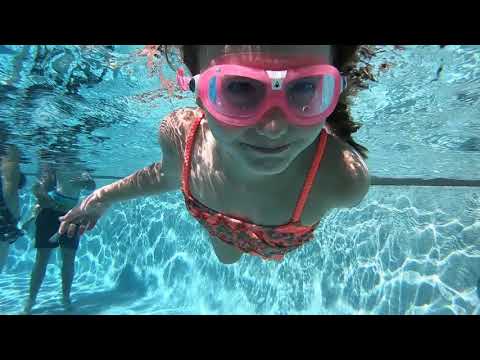This underwater photograph captures a vibrant scene in a swimming pool, featuring a young girl of about 8 or 9 years old, swimming towards the camera with a half-smile on her face. She is wearing pink goggles and the visible part of her two-piece bathing suit is floral with pinkish straps. The crystal-clear water showcases beautiful wave patterns and reflections created by the sunlight. To the left of the girl, the lower bodies of two adults can be seen standing in the pool—one is a man identified by his swim trunks, and next to him is another individual, partly visible, seemingly clad in a one-piece bathing suit. The pool's rounded concrete edges and the walls behind the girl are discernible, enhancing the depth and context of this cheerful, summertime scene.